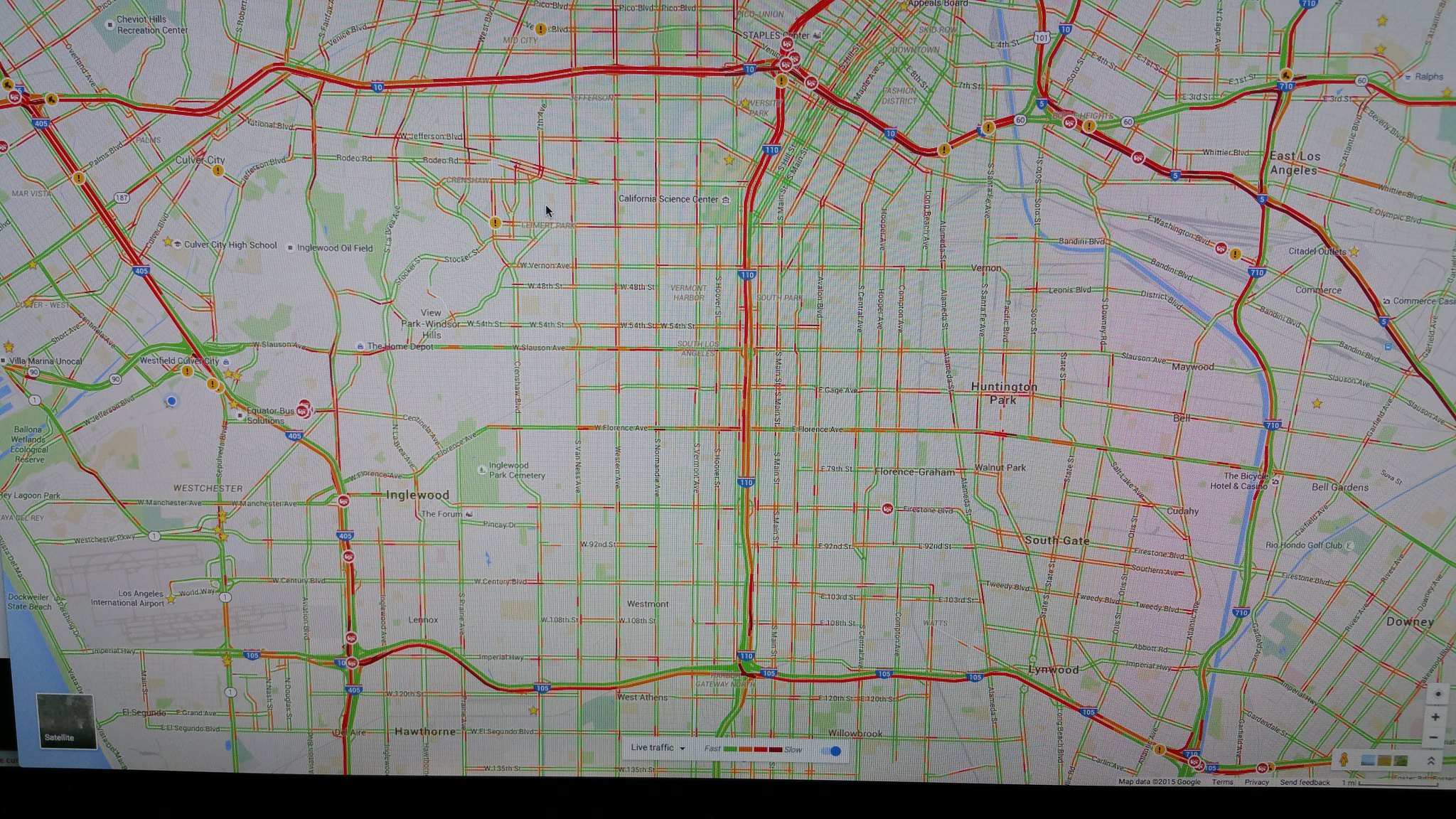This screenshot captures a detailed map, though the text is quite tiny, making the names of cities, roads, and landmarks difficult to decipher. In the lower left-hand corner, a narrow strip of water is visible, suggesting the presence of a small body of water such as a river or a coastal inlet. The layout and markings imply it could be a set of driving directions to an unspecified destination.